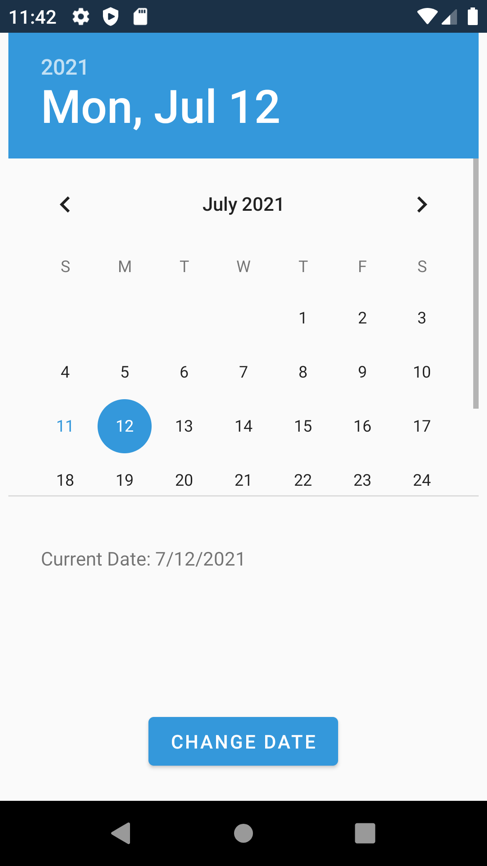This detailed caption accurately describes a smartphone screenshot featuring a calendar app:

"In this smartphone screenshot, the top border is a dark blue containing various status icons: a timestamp reading 11:42, a settings wheel, a shield indicative of virus protection, a calendar icon, a Wi-Fi signal icon, and a battery icon displaying the current charge. 

Directly below the top border, there is a sky-blue banner with white text displaying the date: '2021, Monday, July 12th.' Below this banner is a calendar view for July 2021, with the date '12th' circled in blue to highlight the current day. 

Underneath the calendar, it clearly states 'Current Date: 7-12-2021.' At the bottom of the screen, there is a blue button labeled 'Change Date.' The bottom border of the smartphone screenshot is black and features three grey navigation icons: a left-facing arrow, a home button, and a stop button. This image captures the detailed interface of a calendar app in use on a smartphone."